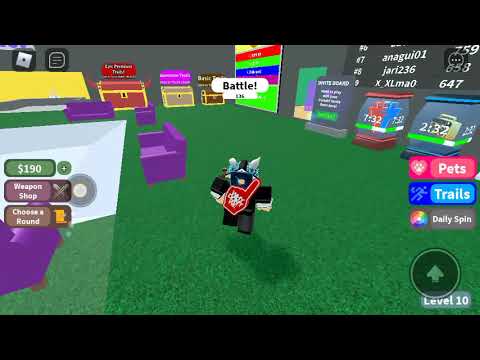The image is a screenshot from a Roblox game and depicts a character-centered scene in a simplistic, blocky 3D environment. The main character, a humanoid cat with square limbs, is adorned in a black outfit, holding a large foam finger with "Why don't we?" inscribed on it. The setting is a green floor with a grass-like texture, indicating it might be an open social area shared by players. Notable elements include purple couches suggesting areas for social interaction, several treasure chests hinting at potential rewards or competitions, and display cases likely meant for trophies.

The interface displays various game options; on the left side, there is a money counter showing $190, along with buttons for a weapon shop and round selection. On the right side, buttons labeled pets, trails, and daily spin provide additional activities for players. This area appears to serve as a hub where players can engage with different features and socialize, with the overall design capturing the essence of a simplistic and communal gaming experience.